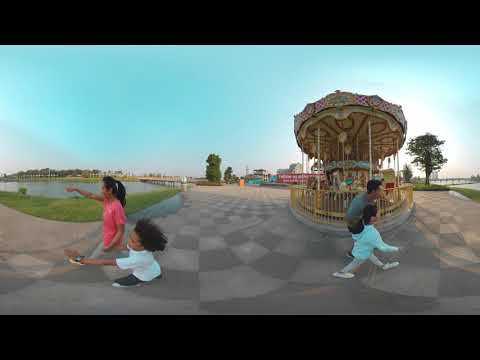The panoramic image, possibly a 360-degree view from a security or monitoring camera, captures a busy scene at a tourist location, likely a fairground or carnival. The scene is split into two apparent sections that might appear spliced together. On the left, a woman with black hair tied in a ponytail is wearing a pink shirt and gray pants. She is walking with a small boy wearing a white shirt and black pants. Both have their arms extending forward as they move leftward. They are strolling on a checkered pattern of tiled paving stones, adjacent to a grassed area and a serene lake under a bright blue, cloudless sky.

On the right side of the image, a man in a gray shirt and black pants is slightly crouched, walking with a young girl in a very light blue shirt and gray pants. Both are heading rightward, in front of a carousel surrounded by a yellow barrier. The background reveals a ferris wheel, sections of greenery, and additional fairground features. The backdrop also features lush trees and more grassed areas, enhancing the vibrant and lively atmosphere of the scene.